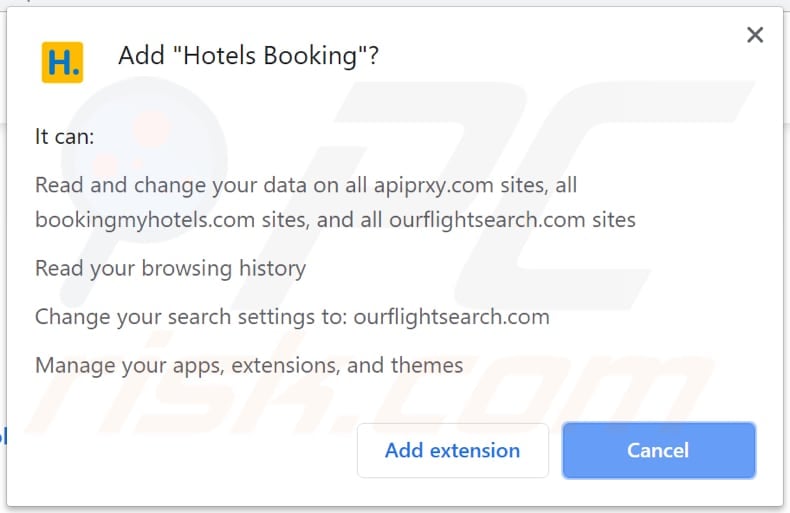This screenshot captures the installation prompt for a browser extension named "Hotels Booking." At the top left, there's a logo consisting of a blue "H" against an orange square, accompanied by a small blue dot at the bottom right corner of the square. Adjacent to the logo, black text reads: "Add 'Hotels Booking'?"

Beneath this header, additional information about the extension's permissions is listed. It states: "It can: read and change your data on all apiprixie.com sites, all bookingmyhotels.com sites, and all our flightsearch.com sites. Read your browsing history, change your search settings to our flightsearch.com, manage your apps, extensions, and themes."

At the bottom right of the prompt, there is a blue button with white text labeled "Cancel." Directly to the left of this button, white text on a blue background reads "Add extension." This setup indicates that the user is being asked to confirm their intent to install the extension on their web browser, such as Google Chrome.